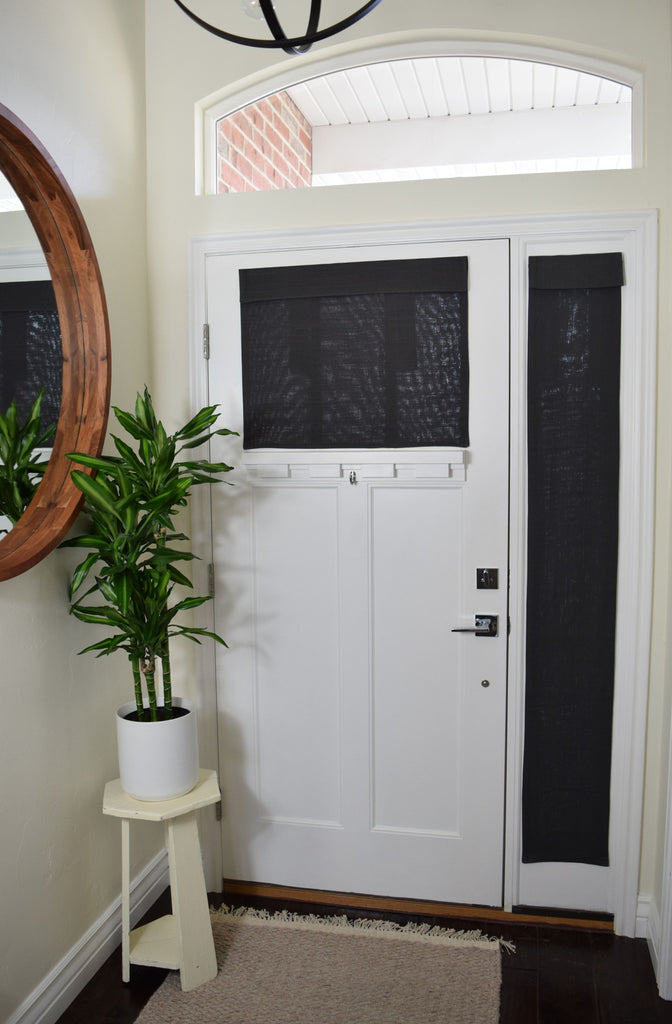This image captures the front entryway of a home, focusing on a white front door set against white walls. The door features a rectangular glass window in the upper part, covered by a black shade, and is equipped with newer silver hardware. To the right of the door, a large rectangular window also has a black shade. Above the door, there is an arched window that provides additional natural light. 

On the floor in front of the door lies a tan rug, which sits atop a black carpet, adding layers to the flooring. To the left of the door, there is a small, modern white table holding a white pot with a green plant that resembles palms. Adjacent to this setup, the left wall adorns a large, circular mirror framed in brown wood. The overall scene is one of modern simplicity, with a mix of practical and decorative elements.